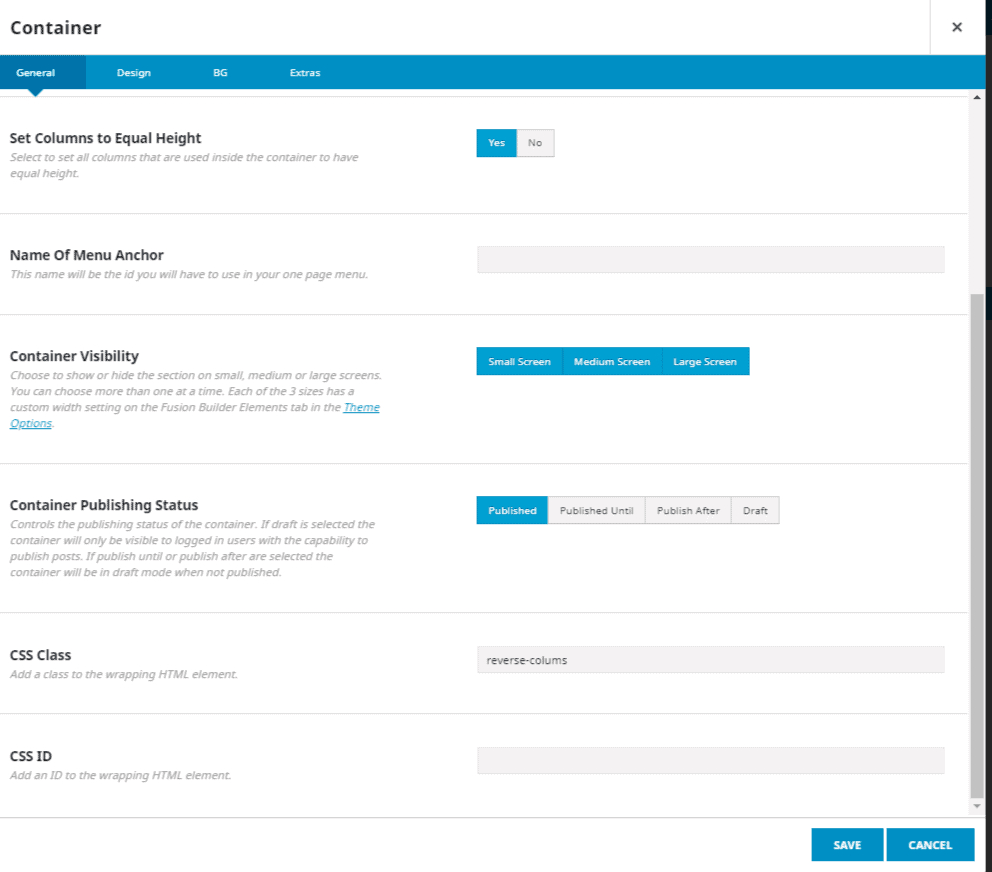Here is the cleaned-up and detailed caption:

"A website screenshot showcasing the container configuration menu in a design tool. The top left corner prominently displays the word 'Container' followed by sub-headings: 'General,' 'Design,' 'BG,' and 'Extras.' An 'X' button is located in the top right corner for closing the menu. The option to 'Set columns to equal height' is present, allowing users to ensure all columns within the container have uniform height. A 'Yes' option is highlighted next to this feature.

Below, there's an informational section about the 'Name of menu anchor,' indicating that the provided name will function as the ID for the one-page menu. A text field awaits user input here. The 'Container visibility' section comes next, allowing users to control the section's visibility across small, medium, or large screens, with the flexibility to select multiple sizes simultaneously. These options are highlighted in blue.

The 'Container publishing status' section controls whether the container is published or in draft mode. If 'Draft' is selected, only users with publishing capabilities will see the container. Blue highlights the 'Publish' option, while other options are grayed out.

Additional settings include fields for adding a 'CSS class' and 'CSS ID' to the HTML element, with 'Reverse columns' being selected. The section concludes with 'Save' and 'Cancel' buttons at the bottom, with the 'Save' button highlighted in blue."